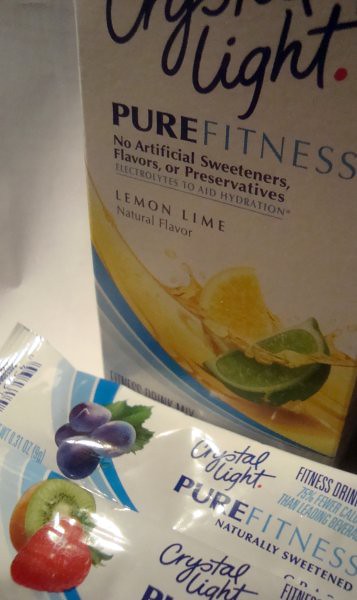The image depicts a close-up shot of a Crystal Light product, specifically showcasing the lower half of its box alongside two individual beverage mix packets. The box prominently displays the branding "Crystal Light Pure Fitness" and highlights key product attributes such as "No Artificial Sweeteners, Flavors, or Preservatives" and "Electrolytes to Aid Hydration." The flavor detailed on the box is "Lemon Lime Natural Flavor," illustrated with vibrant imagery of a lemon and a lime immersed in a yellow liquid. Positioned in front of the box are two distinct Crystal Light Pure Fitness packets. One packet features a blueberry graphic, suggesting a blueberry flavor, while the other packet, though partially cut off, displays images of a kiwi and a strawberry, indicating a kiwi-strawberry flavor. The combination of these visual elements emphasizes the product's natural and fitness-oriented branding.